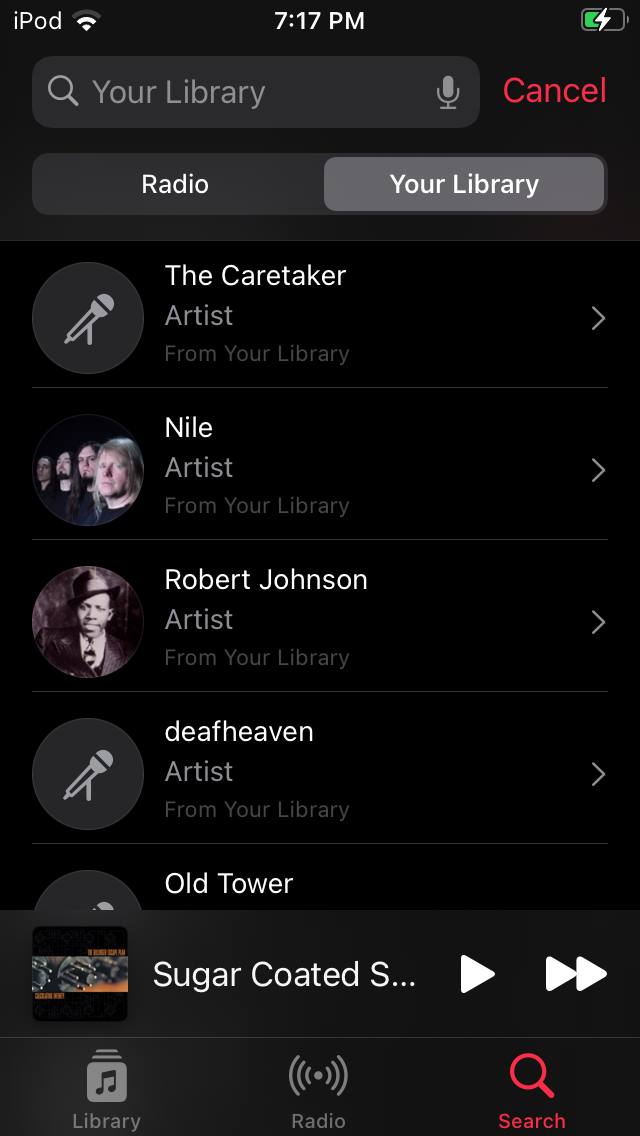In the image, the interface of a music application is being displayed. At the very top, there is a search bar accompanied by a magnifying glass icon, labeled "Your Library." Right next to the search bar, there is a microphone logo and a red cancel button. Below the search bar, there are two tabs labeled "Radio" and "Your Library," with "Your Library" being the selected tab.

The screen shows a list of songs and artists from the user's library. The first entry is a song titled "The Caretaker" with an artist labeled as 'artist', but it lacks album art, represented by a gray circle with a microphone. Following this is Niall, another artist from the user's library; their entry includes an image of the band members looking off camera. Next is Robert Johnson, a notable artist in the library, accompanied by a black-and-white photograph of a man in a suit, likely of African American descent. Following is Deaf Heaven, another artist from the library, which, like 'The Caretaker,' lacks album art and is represented by the gray circle with a microphone icon. The final visible entry is Old Tower, although its details are cut off.

At the bottom of the interface, there is a navigation bar with three tabs: "Library" (depicted as a stack of boxes with a music note), "Radio" (depicted with a radio wave symbol), and "Search" (indicated by a red magnifying glass icon).

Notably, the time displayed at the top center of the screen reads 7:17.